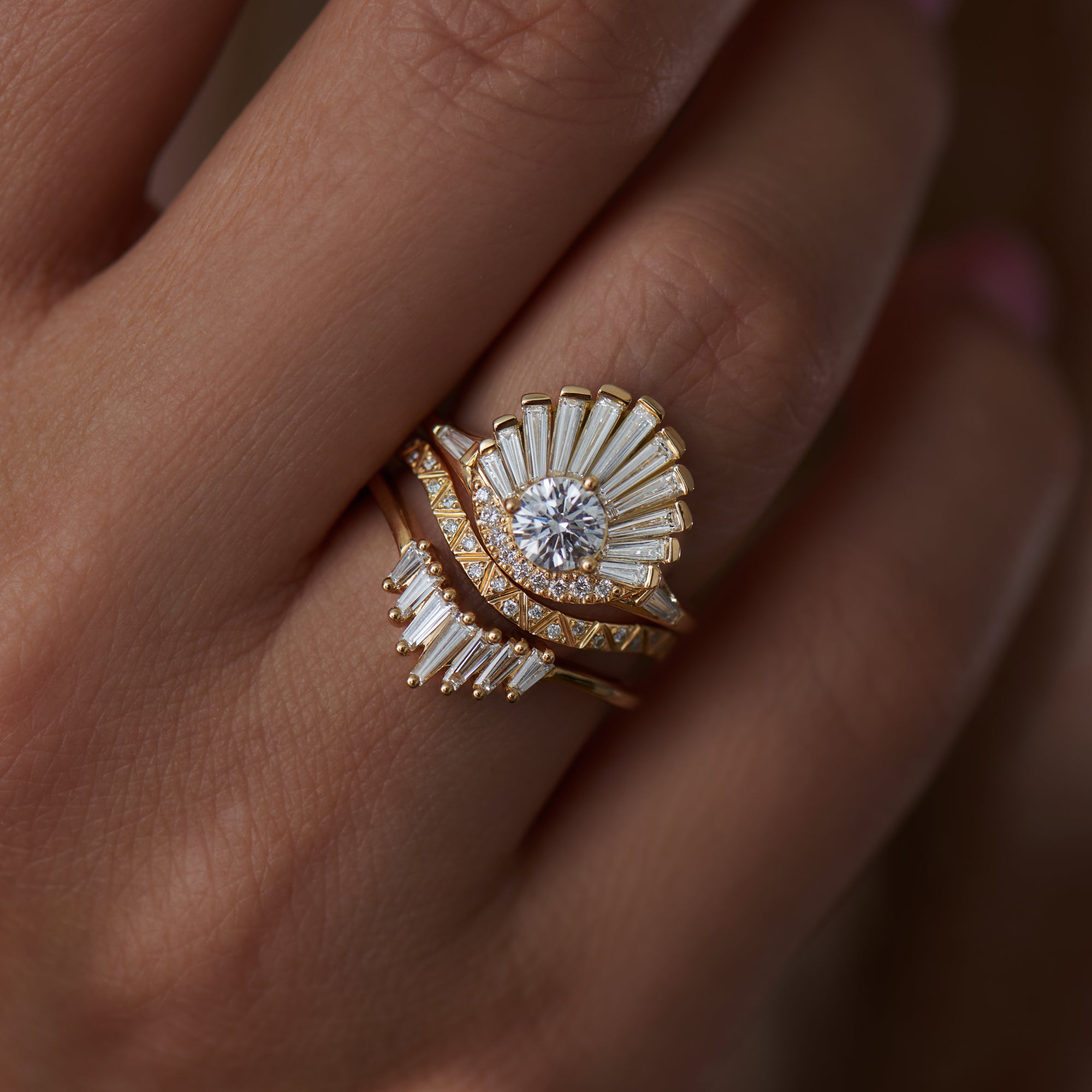This is an intricate close-up image focusing on the middle finger of a Caucasian woman's hand adorned with a very ornate and decorated gold ring. The photograph highlights the detailed creases and wrinkles of the skin, from the knuckles almost to the fingernails, revealing three fingers. The middle finger showcases a striking gold ring featuring a central diamond surrounded by a semicircle of petal-like, clear jewels, giving a sunray appearance. Below the diamond setting, the ring displays an elaborate gold design interspersed with small strips of diamonds flanked by tiny gold beads, creating a rich, almost multi-layered effect. The hand also sports pink nail polish visible on one finger, adding to the overall elegance of the composition.